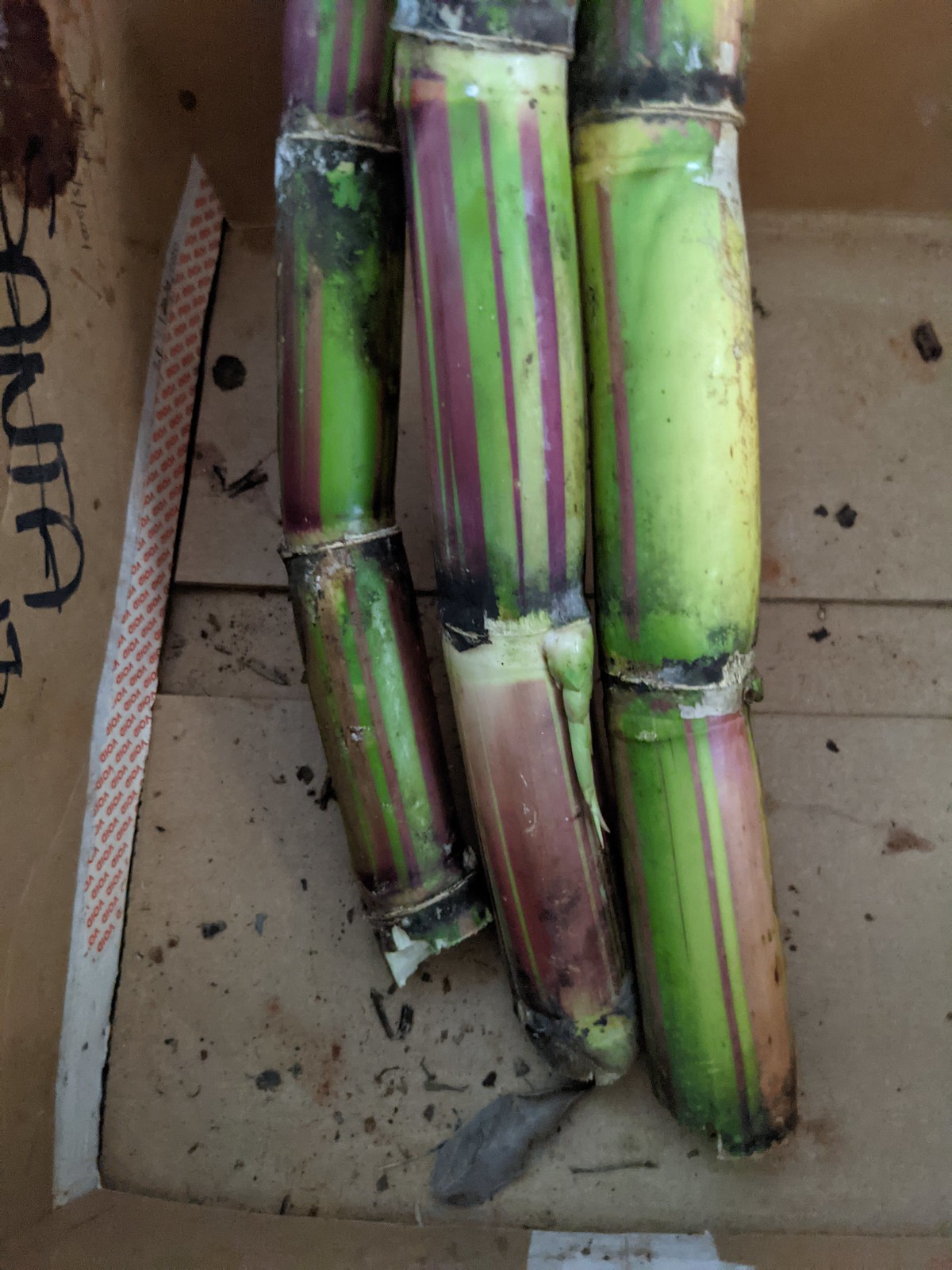This photograph features a close-up of three sugar cane stalks nestled inside a cardboard box. The stalks are primarily a bright grasshopper green, interspersed with maroon, violet, and light purple stripes, giving them a unique, almost rhubarb-like color pattern. Each stalk exhibits multiple joints, showing off segments and thick green roots beginning to grow from the center stalk. The joints on the stalks are marked with black smudges. At the bottom of the box, there are traces of dirt and some debris, including leaves and black dots. On the left side of the cardboard box, there is writing in black magic marker, partially legible with the word "Santa." Additionally, a small piece of paper with illegible writing lies at the bottom, and a white sticker with red lettering is visible on the right side.